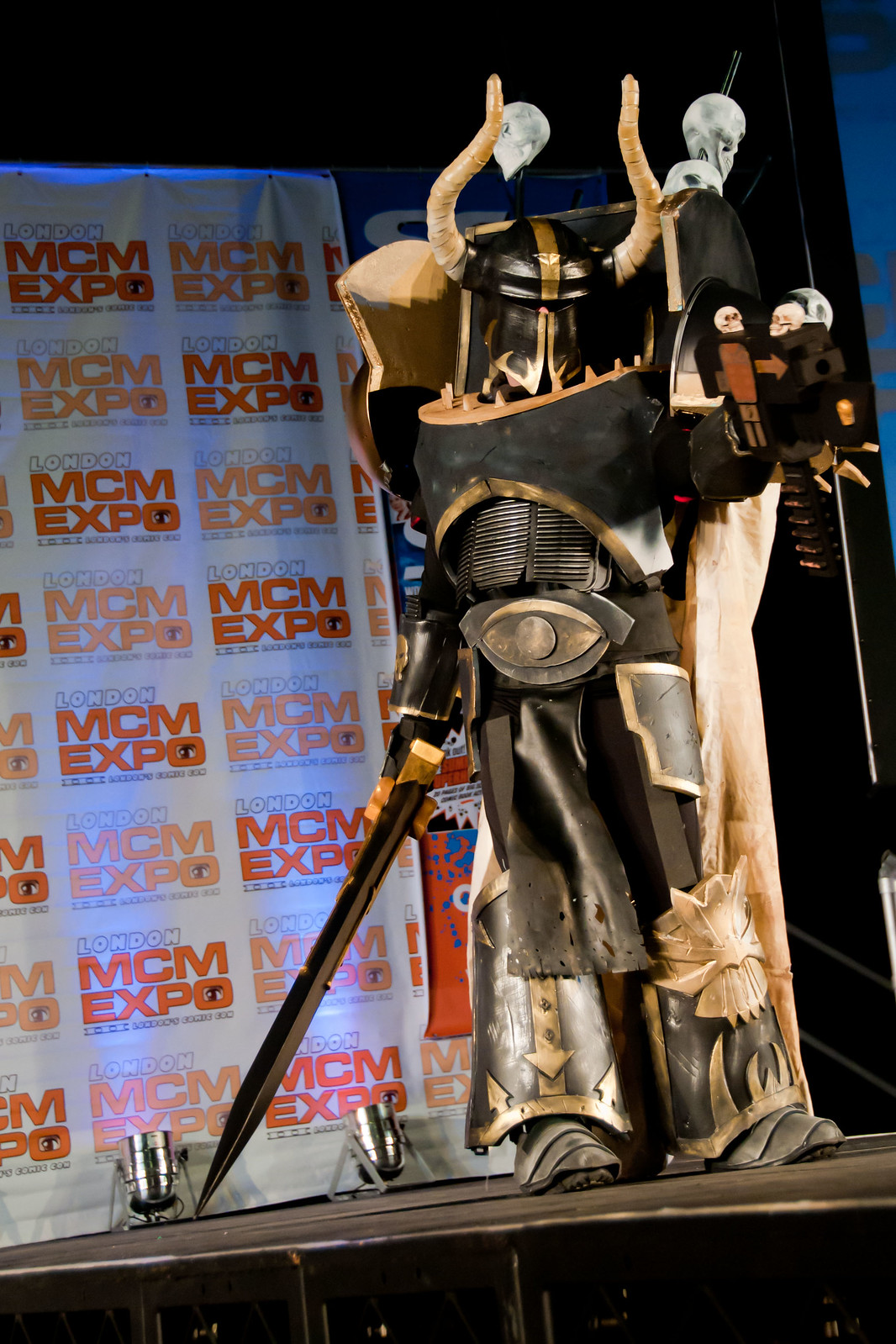The photograph captures a detailed costume at an indoor convention, likely the MCM Expo in London, as indicated by the background banners. It features a person in an elaborate, fantasy-inspired armored outfit, reminiscent of a digital game or comic book character. The individual stands on a black stage beneath a canopy of hanging skulls. Their armor includes exaggerated, gold-accented black leggings and a matching breastplate, complete with flames details. A cream-colored cape flows down their back. The character wears a black helmet with eye slits, a yellow line down the center, and two prominent golden horns. Their face is fully obscured by the helmet. In their left hand, they hold a long sword that touches the stage. The ensemble also features a unique belt with a football-shaped buckle, and the person sports gray boots. This striking costume, blending elements of a samurai and a futuristic warrior, showcases intricate craftsmanship and adds to the vibrant, fantastical atmosphere of the expo.